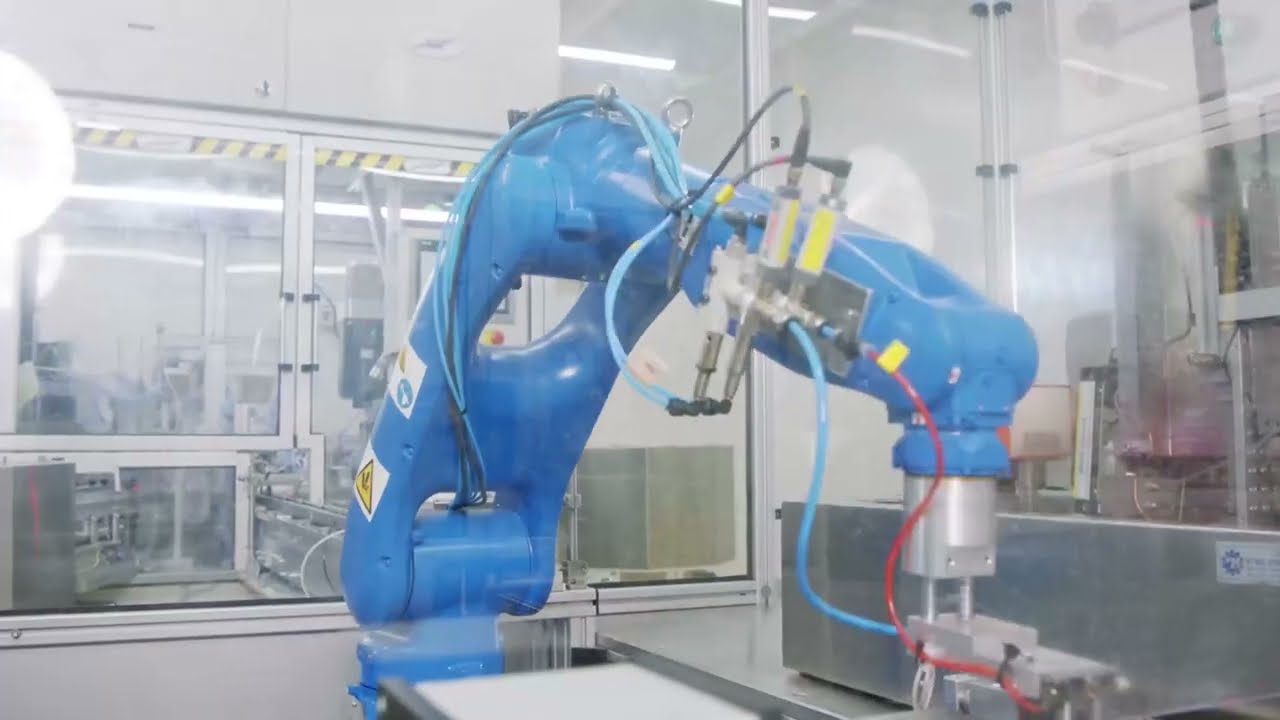The photo captures an intricate blue robotic arm situated in a spacious factory or industrial setting. The arm, which seems to be a critical component of an assembly line, is equipped with multiple tubes—primarily blue and red—that resemble paint dispense systems. Some of these tubes are attached to brush-like tools, hinting that the machine might be involved in painting or applying coatings. The large, robust arm is stationed in an environment characterized by gray and white tones, surrounded by large windows with aluminum framing that illuminate the space with natural light. High above, fluorescent lights add to the industrial ambiance. Warning tapes and caution patches are visible at various points, underscoring the machine's powerful and potentially hazardous nature. To the right of the arm, a section of the wall and a door can be seen, further indicating the factory's expansive layout which includes more machinery visible through additional windows. This elaborate setup suggests a specialized use that requires experienced operators, possibly in the manufacturing or heavy machinery production sector.